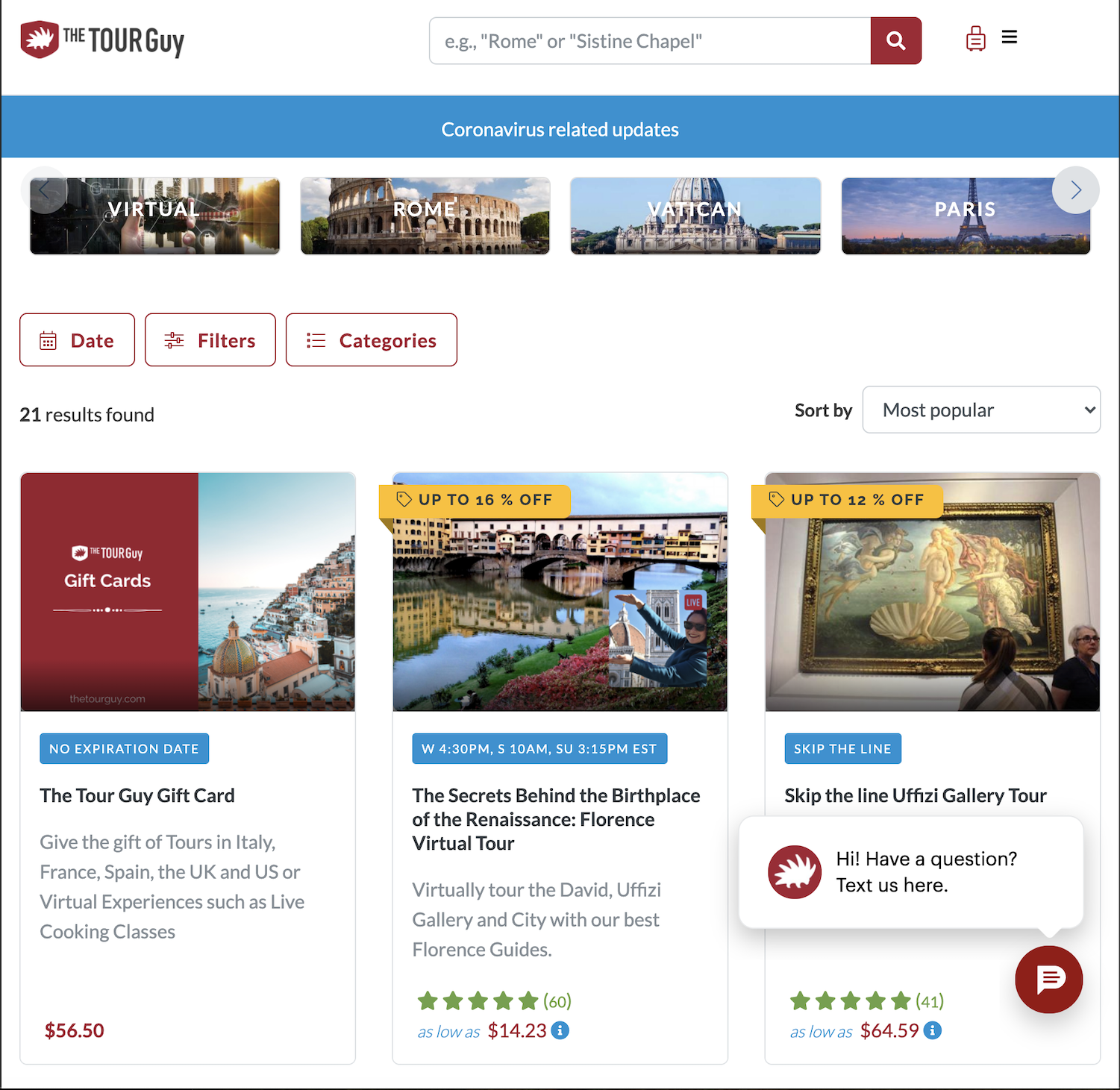A detailed screenshot of "The Tour Guide" website is showcased, a platform offering various purchasable tours. At the very top of the page is a search bar featuring a placeholder text "e.g., Rome or Sistine Chapel," accompanied by a magnifying glass button for initiating a search. Adjacent to the search button, a luggage icon with three horizontal lines indicates additional settings or options.

Below the search bar, there is a prominent blue banner providing coronavirus-related updates. Further down, a series of clickable square buttons represent different types of tours, arranged horizontally. From left to right, the options are labeled as "Virtual," "Rome," "Vatican," "Paris," followed by an arrow hinting at more options available upon clicking.

Beneath these buttons, there are labeled sections for "Date," "Filters," and "Categories," each represented by clickable buttons. The interface indicates there are "21 results found," with a sorting option available. Presently, the list is sorted by "Most Popular," as shown in a drop-down box.

Further down, a promotional banner advertises a "Tour Guide Gift Card," highlighting the opportunity to give the gift of tours across Italy, France, Spain, the UK, and the US, or to engage in virtual experiences like live cooking classes, priced at $56.50. Additionally, two featured tours are promoted: "Secrets Behind the Birthplace of the Renaissance: Florence Virtual Tour" and "Skip the Line Uffizi Gallery Tour."